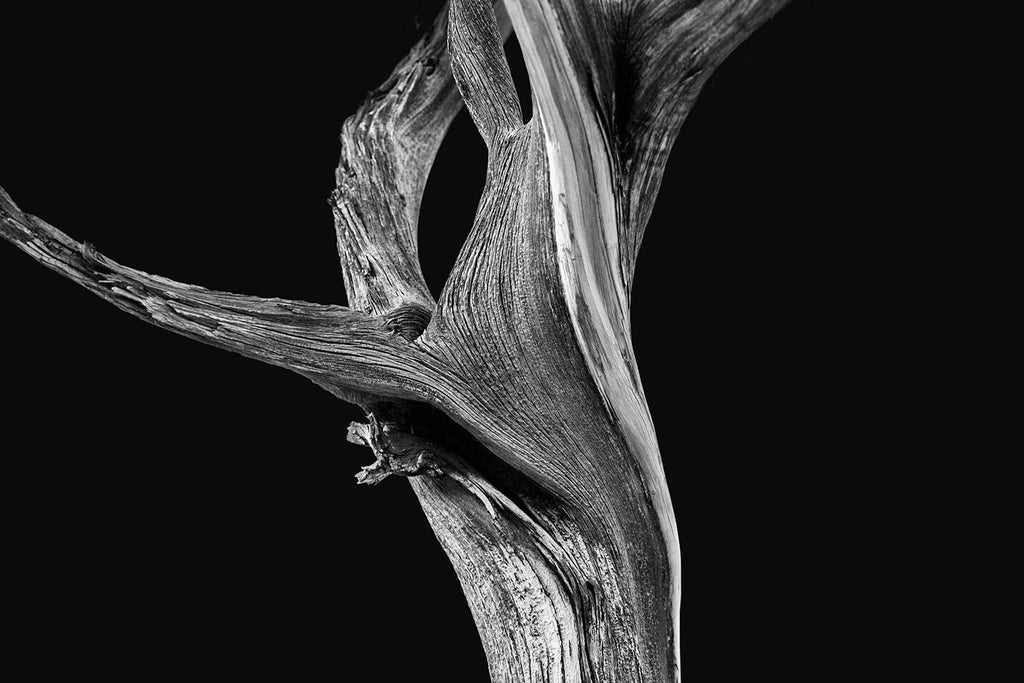In this black and white photograph, the majority of the background is a solid, deep black, creating a stark contrast with the central subject of the image. Dominating the scene is an abstract, twisted form reminiscent of a tree trunk with multiple branches. Starting from a thicker base at the bottom, the image features a knotted section of the wood and a broken branch jutting out to the left. From the middle, two main branches ascend upward and diverge into further smaller, twisted segments, one path heading to the left and the other to the right. The intricate play of light and shadow highlights the white bark textures and reveals shaded areas, adding depth to the otherwise simplistic yet evocative scene. A small hole is noticeable near the bottom left, contributing to the natural, weathered look of the subject. Overall, the photograph captures the intricate, splintering pattern of the tree-like structure against a pure black backdrop, presenting a hauntingly beautiful and ambiguous image.